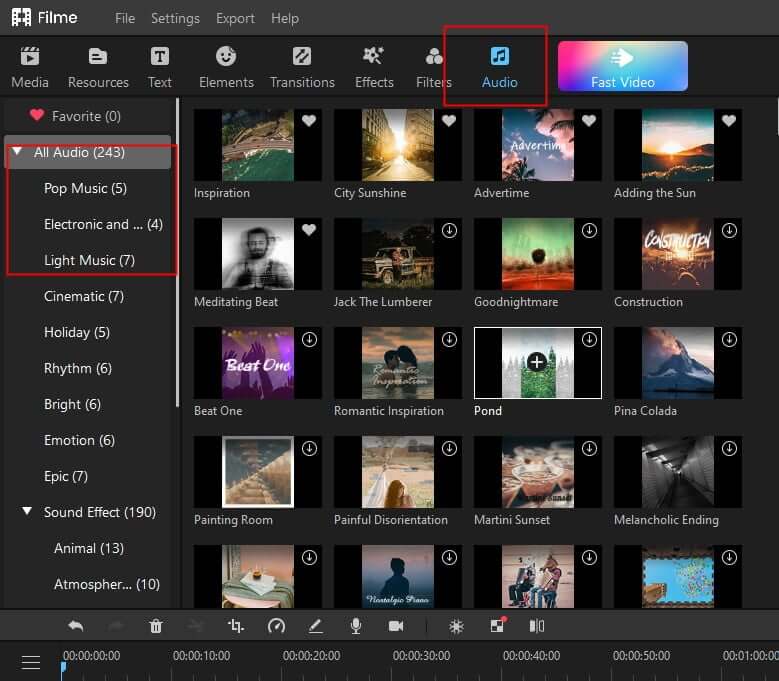This image is a screenshot from a media library interface, showcasing a collection of music albums. The entire background is black, and numerous small squares representing album covers are neatly organized on the screen. Each square contains a distinct album cover image, indicating that the collection encompasses various musical genres.

On the left side of the image, there is a vertical navigation bar highlighted in a red silhouette style, listing categories such as "All Audio," "Pop Music," "Electronic," "Light Music," "Cinematic," "Holiday," "Rhythm," "Bright," "Emotion," "Epic," "Sound Effect," "Animal," and "Atmosphere." 

Within this selection panel, certain albums have icons displayed over them: a solid heart icon signifies favorites, while a download icon indicates availability for download. Additionally, each album comes with a visible duration label, specifying the length of each track.

Among the albums, partial titles such as "Painting Room," "Painful," "Disoriented," "Martini Sunset," and "Melancholic Ending" can be discerned, hinting at the nature and mood of the tracks they contain. The interface presents a grid of 4x5, amounting to a total of 20 albums visible within this screenshot.